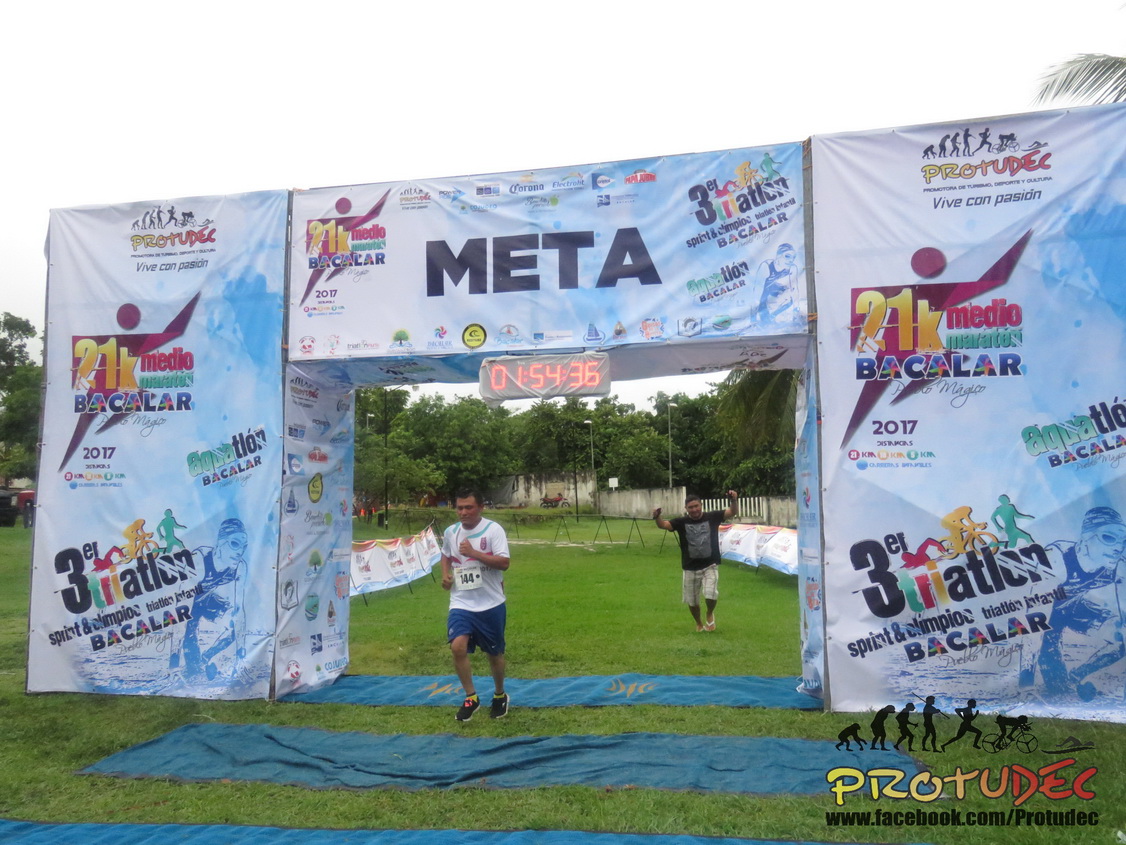The photograph captures a dynamic moment at the finish line of a race, framed by a large, boxy arch structure inscribed with the bold text "META" at the top. This arch serves as the official marker for the race's conclusion and features various sponsorship logos and words such as "triathlon," "sprint," "champion," "baccalaureate 2017," and "vive compassion." Below "META," a timer reads 1 hour, 54 minutes, and 36 seconds. The event takes place outdoors under a gray, overcast sky. Two men are crossing the blue carpet runner that leads to the finish line; the foreground runner wears blue shorts, white shirt, and sneakers, with an obscured race number, while the man behind him, also nearing the finish, sports a black short-sleeve shirt and dark shorts, celebratory with arms raised. The terrain beneath the carpet runner is grassy, and additional branding, including "Pro2Deck" and a Facebook URL, is visible in the lower right corner of the image.